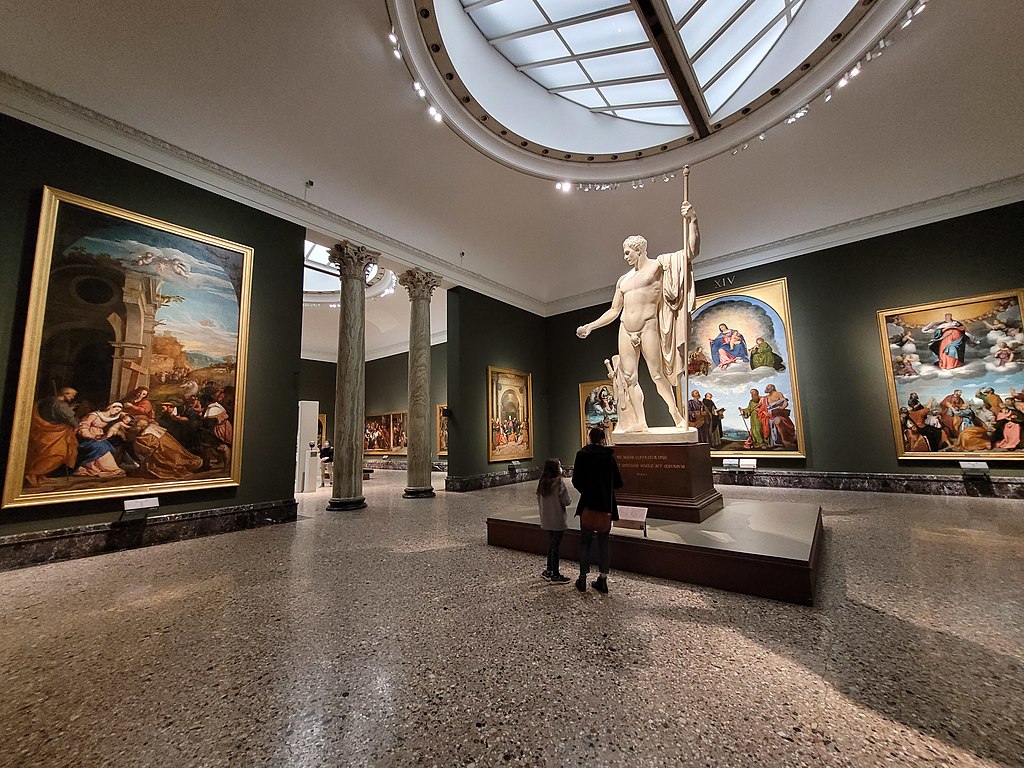In the center of a grand art gallery with a large marble floor and a domed skylight flooding the space with natural light stands a striking 15-foot-high marble statue of a nude man. The statue, reminiscent of classical Greek art, holds a sphere in his outstretched arm and has a draped cloak over his left arm. It is set atop a sturdy pedestal, capturing the attention of a woman and her young daughter, who are closely reading the inscription at its base.

The gallery's ornate interior features white, yellow, gold, red, and purple hues. Framing the scene are imposing columns that add to the room's grandeur. The left walls showcase depictions of medieval settings while the back walls are adorned with grand Renaissance and religious paintings, each encased in gilded frames and many of colossal scale—most are at least six feet tall and wide. The museum's highly polished terrazzo floor and fisheye lens effect in the photograph accentuate the vastness and opulence of this cultural haven.